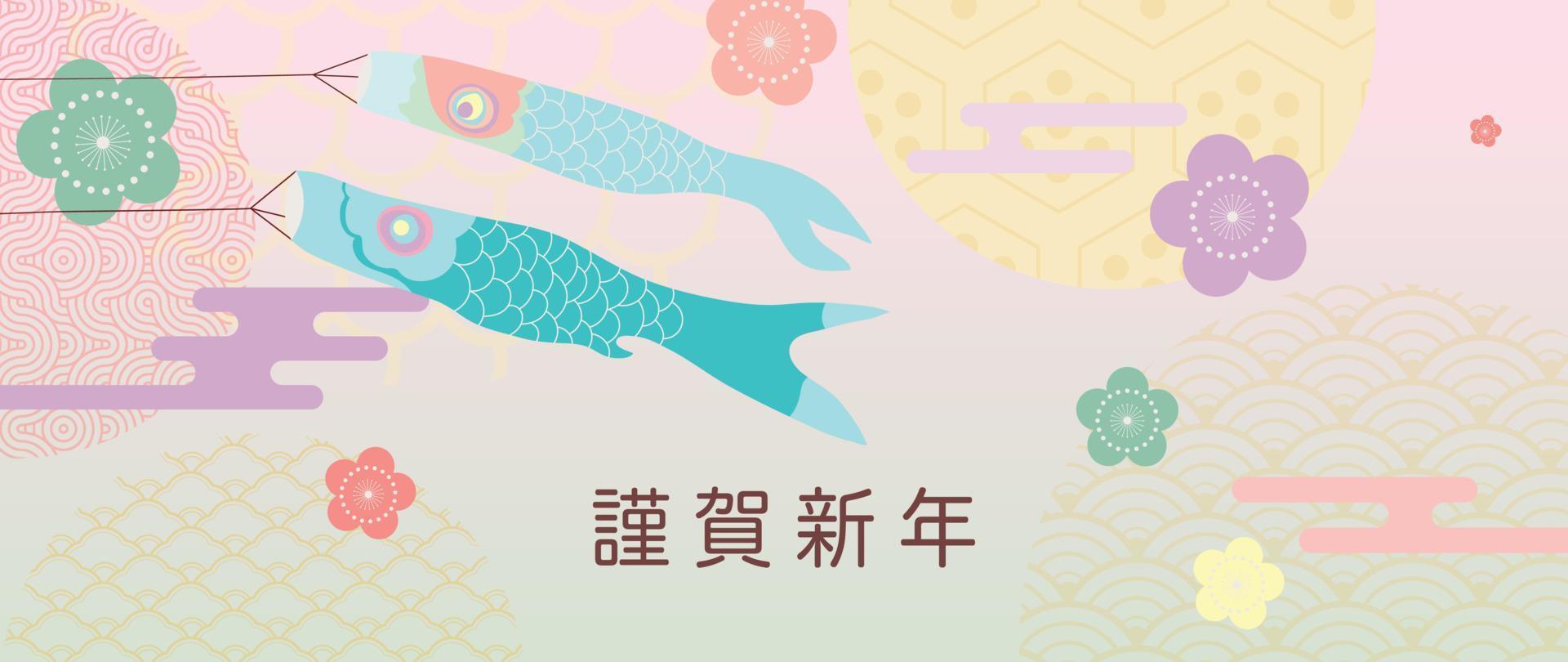This whimsical, rectangular graphic features a playful scene of two fish kites floating gracefully, with strings trailing as if they're flying through the sky. The kites, one light blue and the other teal with details around their eyes, emerge from the left side of the composition, their tails fluttering in the breeze. The background is a delicate light pink with intricate Japanese wave patterns resembling fish scales or partial rainbows layered to create a sense of motion. Scattered throughout the image are various flowers in hues of purple, pink, green, yellow, and red, adding vibrant pops of color. Some of the flowers feature basic shapes, with a notable green five-petal flower at the top left, and others arranged more centrally. The bottom part of the image is a soft light yellow with a subtle grid-like pattern, and it is adorned with maroon Japanese characters. Additionally, hexagon and octagonal icons accent the design, giving it an even more dynamic and lively feel.